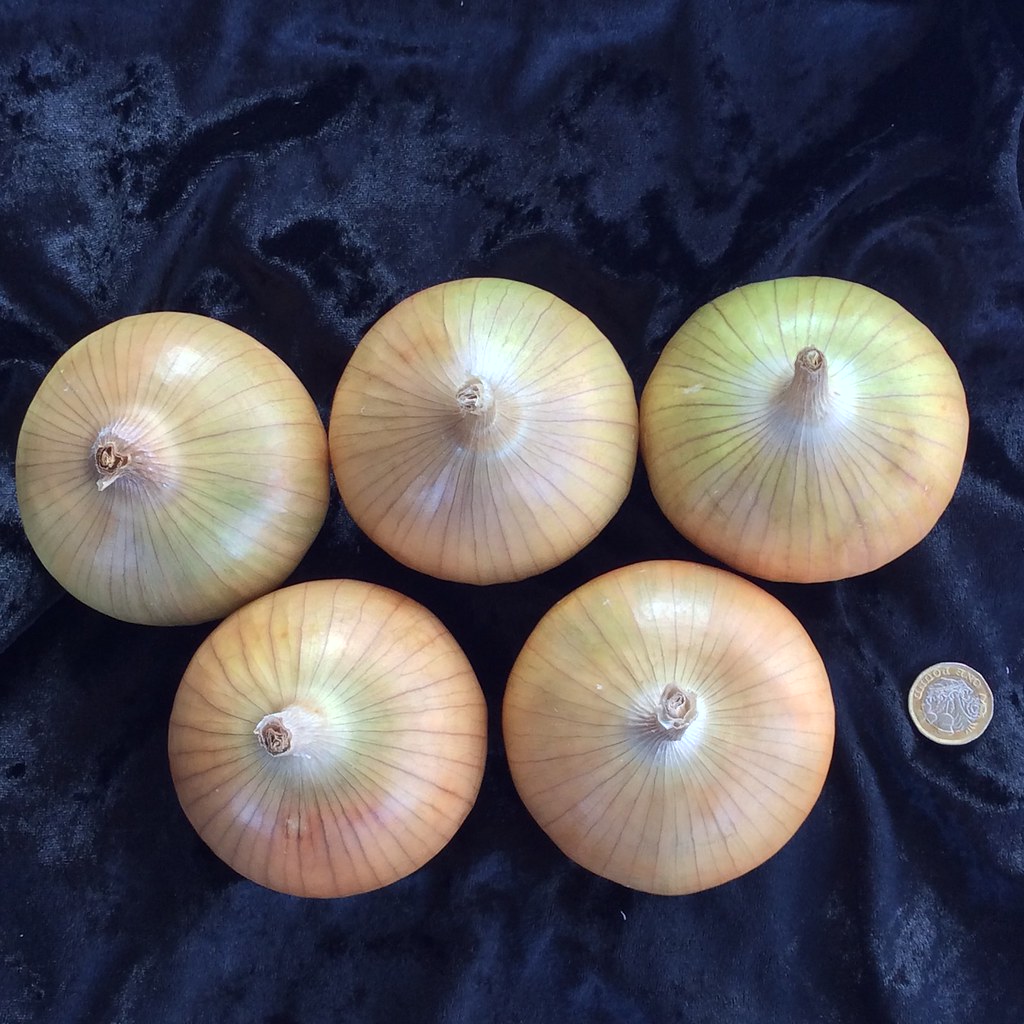In this overhead photograph, a distinct arrangement of five unpeeled onions is captured on a dark, navy blue velvet cloth. The cloth is slightly wrinkled and bunched up in areas, creating shadowy, darkened sections. The onions, exhibiting a healthy and fresh appearance with light brown skins, are arranged in an Olympic pattern—three across the top row and two on the bottom row. Each onion’s trimmed stem is visible from this top-down view. Beside the two onions in the bottom row lies a single, nondescript coin. Its copper hue, coupled with some faint etchings, adds an intriguing element to the composition, though its design is indistinct. A soft light casts a subtle reflection on the onions, enhancing the textured contrast of their skins against the rich velvet backdrop.